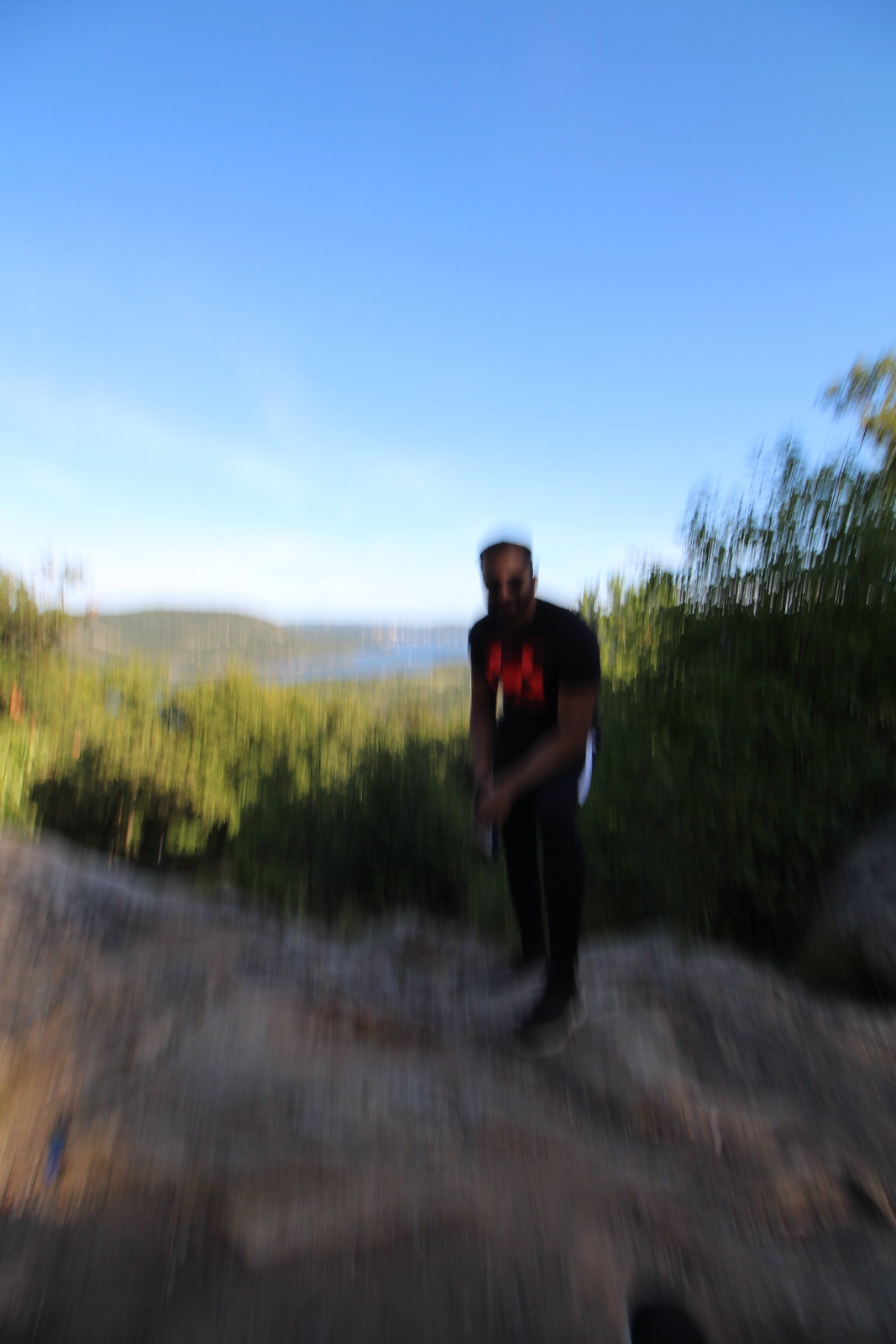In this photograph taken outdoors, a man with a medium complexion stands atop a rocky bluff, surrounded by the natural beauty of the landscape. He is dressed in a black t-shirt adorned with a red logo on the chest, black pants, and gray boots. His look is completed with dark sunglasses. The clear blue sky above is dotted with a few sparse white clouds near the horizon. In the distance, low rolling green hills and a waterway, likely a bay or river, reflect the sky, while lush, sunlit trees add vibrant greenery closer to the camera. The man strikes a casual pose, leaning with his forearm on his knee, as the sunlight casts a warm glow over the scenery.